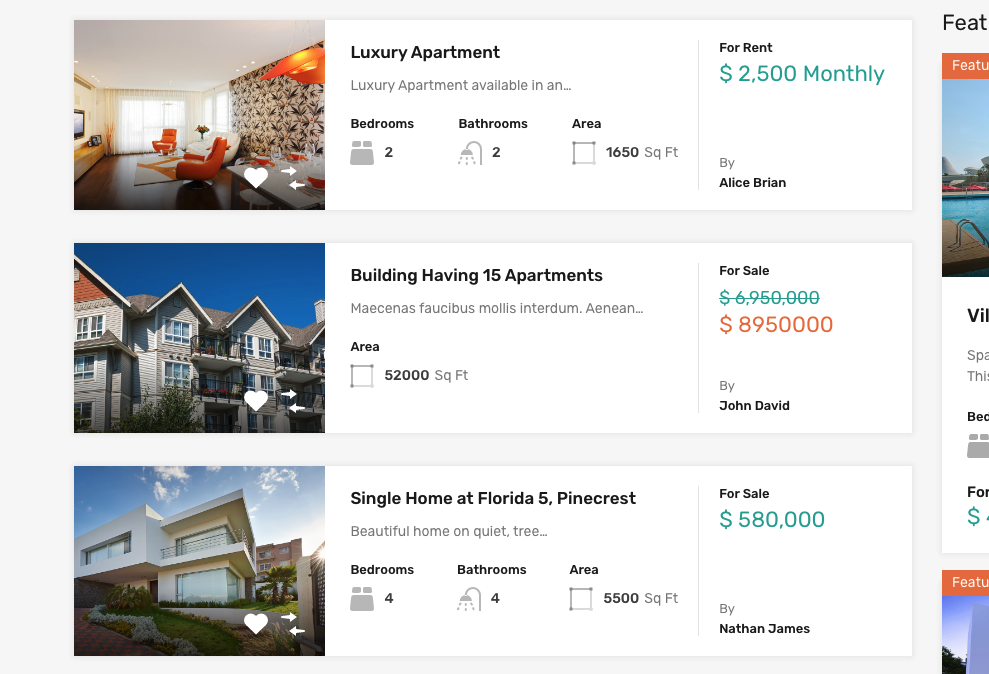In the screenshot, a person is browsing a real estate research website in search of apartments. The image displays several property listings at the top, starting with a luxury apartment adorned with a leaf-patterned wallpaper and two large orange armchairs. This luxury apartment offers two bedrooms, two bathrooms, spans 1,650 square feet, and is available for rent at a price range of $2,500 to $2,500 monthly.

Following this, there is a listing for a building comprising 15 apartments, covering an area of 52,000 square feet, which is on sale for $8.95 million, represented by John David. Additionally, there’s a listing for a single-family home located in Pinecrest, Florida, featuring four bedrooms and four bathrooms, spread across 5,500 square feet, with a price tag of $580,000, listed by Nathan James. The overall scene indicates that the individual is actively seeking a place to live.